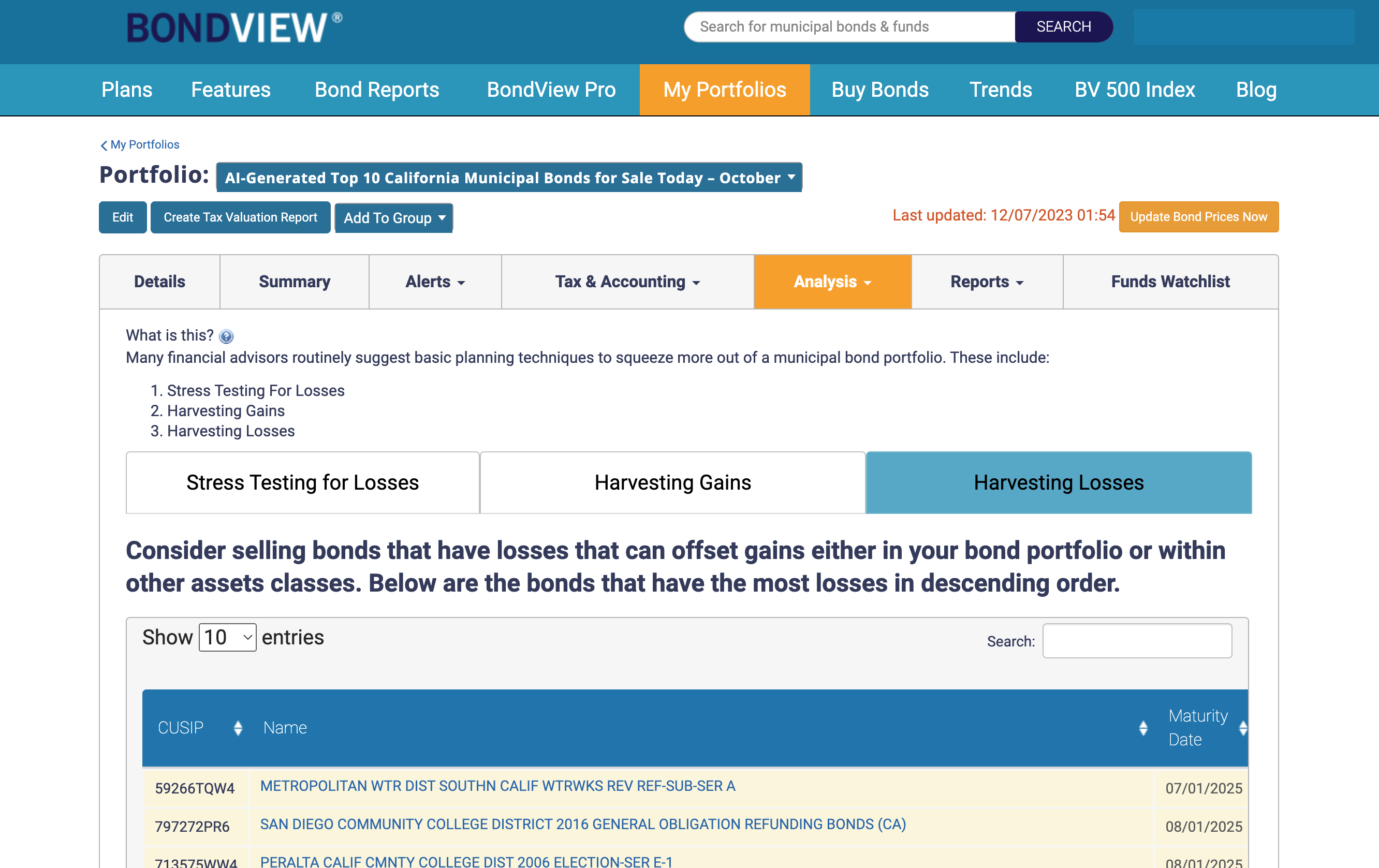The image is a screenshot of a website's portfolio section, specifically titled "BondView." At the top left corner, the BondView logo is visible. Below the logo, there are multiple navigation tabs, with the current view emphasizing the "My Portfolios" tab.

On the left sidebar, there is a section labeled "Portfolio: AI Generated Top 10 California Municipal Bonds for Sale Today October." Underneath, it highlights the selected sub-tab, "Analysis." 

In the central workspace of the page, another tab titled "Harvesting Losses" is chosen. This tab provides investment advice with the instruction: "Consider selling bonds that have losses that can offset gains either in your bond portfolio or within other asset classes. Below are the bonds that have the most losses in descending order."

The first bond listed is the "Metropolitan WTR District Southern California Revenue" bond with a maturity date of July 1, 2025.